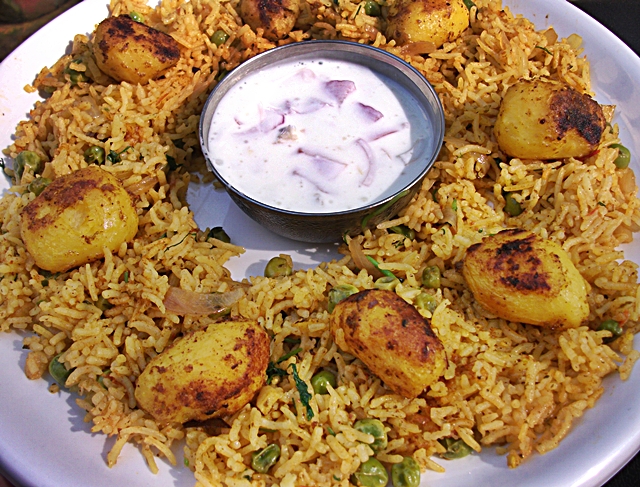This is a detailed, color photograph showcasing a culinary presentation on a round white plate, although the plate's edges are slightly cropped. The main feature is a ring of seasoned, reddish-yellow rice mixed with green peas and possibly topped with chunks that could be either roasted potatoes or chicken. This ring is meticulously arranged to form a wreath-like shape around a central small silver ramekin bowl. The bowl contains a white, creamy liquid, which appears to be either yogurt or milk, and is garnished with slices of red onion. This intricate dish combines vibrant colors and textures, creating a visually appealing and appetizing presentation.